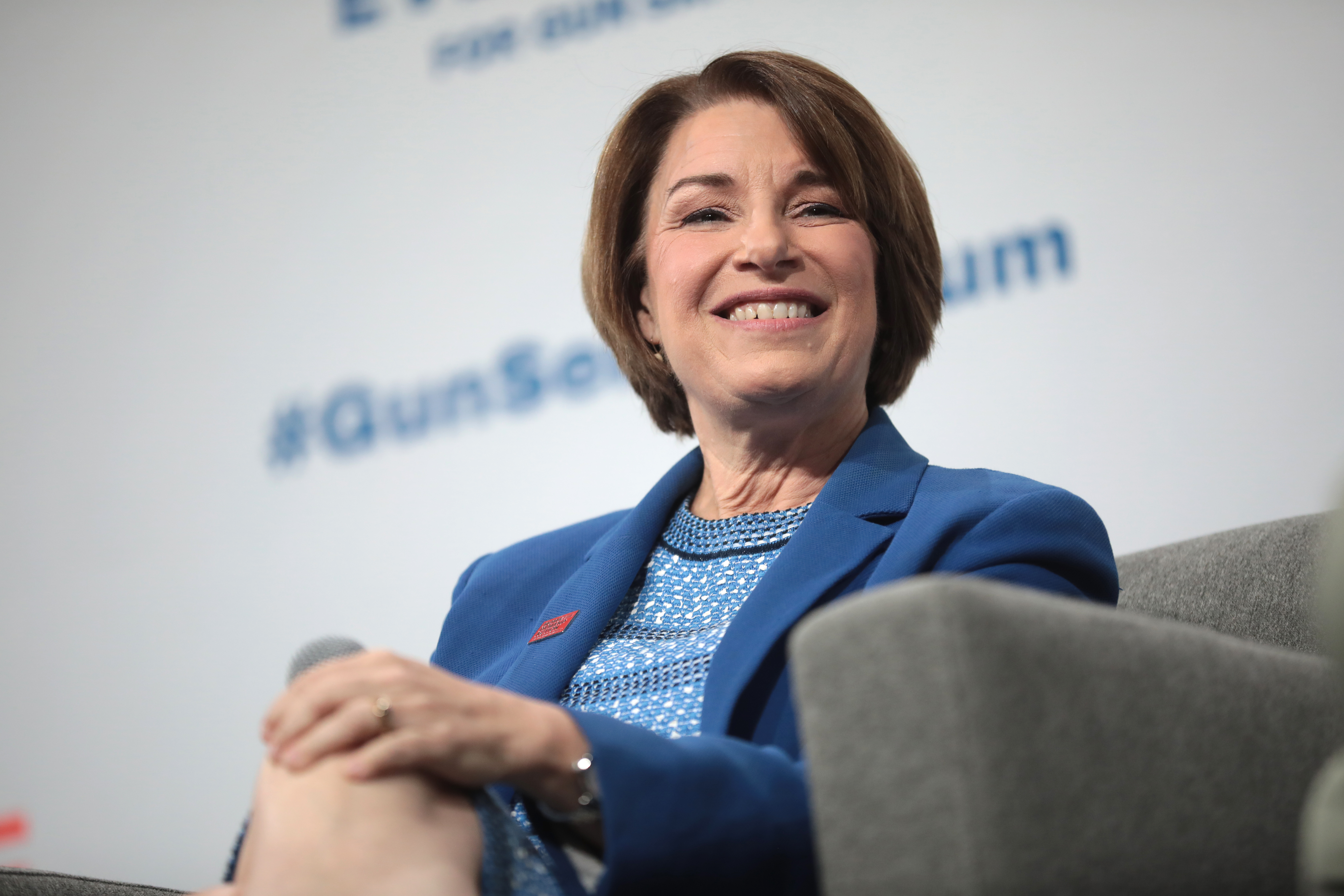This image captures Amy Klobuchar, the senator from Minnesota, in a relaxed, candid moment. She’s seated on a gray, felt-like couch or chair, appearing to be at a public event or forum. Klobuchar is smiling warmly and looking slightly off-camera, perhaps engaging with someone nearby or addressing an audience. She wears a neatly styled, short dark hairstyle and a blue suit jacket over a multi-shaded blue and white, lined and dotted blouse. Her left hand, adorned with a watch partially hidden by her sleeve and a ring on her ring finger, rests comfortably on her crossed knee. In the background, a partially obscured white banner or board with blue lettering hints at the formal setting. The shot is taken from a lower angle, suggesting it might be from the stage's edge, adding to the dynamic composition.